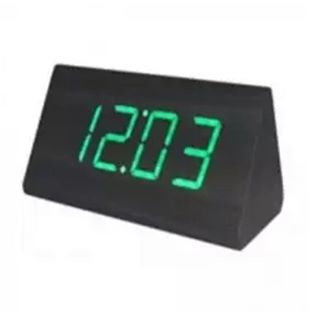The image features a detailed 3D model of a digital clock rendered against a pure white or transparent background, giving it a floating appearance. The body of the clock is black and forms a rectangle when viewed from the front and a triangle from the side, with the right-hand side fully visible. The time displayed on the clock is 12:03, with green digital numbers composed of segmented parts typical of digital displays. The numbers include a one, followed by a two, two dots vertically aligned (colon), a zero, and a three. The clock face is designed to slope slightly upwards due to its triangular shape, indicating it is likely a graphic created for a video game or a digital animation.